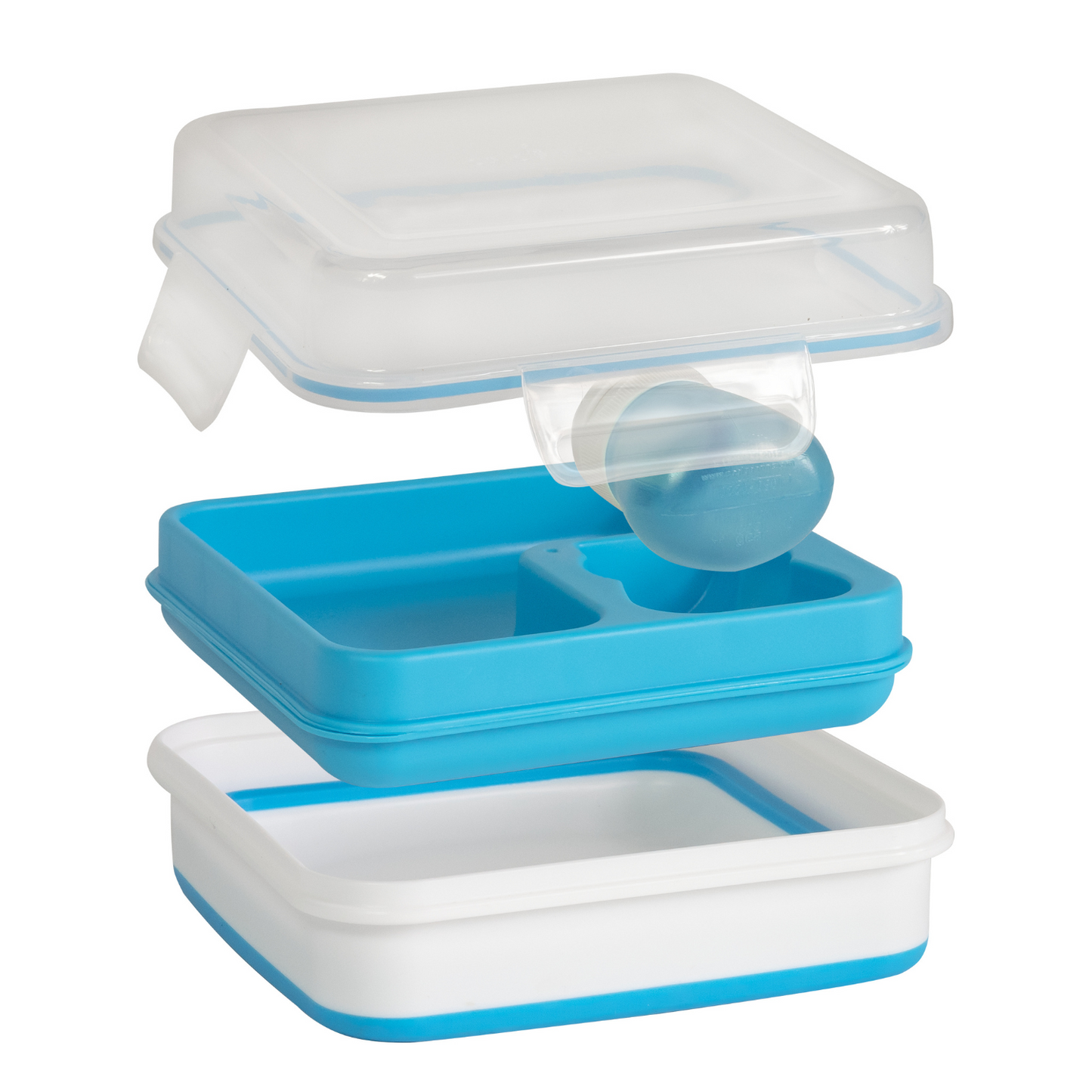The image depicts an exploded view of a bento-style lunchbox against a plain white background, showcasing its individual components suspended as if floating in space. The base of the container is a white Tupperware-style box, measuring approximately four by six inches and standing an inch and a half tall, with a distinctive blue rim around the bottom. Within this base sits a removable blue insert that features three compartments — one large section and two smaller ones. This insert is designed to be filled with water and frozen, thereby keeping the contents cool throughout the day. Nestled perfectly into one of the smaller compartments of the insert is a small squeeze bottle, presumably meant for condiments or salad dressing. Capping off the assembly is a clear, slightly translucent lid equipped with a blue gasket to ensure a tight seal, along with four latches that snap securely onto the base. An additional element shaped like a blue and white punching glove, which may hint at a playful design or branding, is positioned underneath the lid. This comprehensive design makes it an ideal lunch kit, particularly suitable for school children.